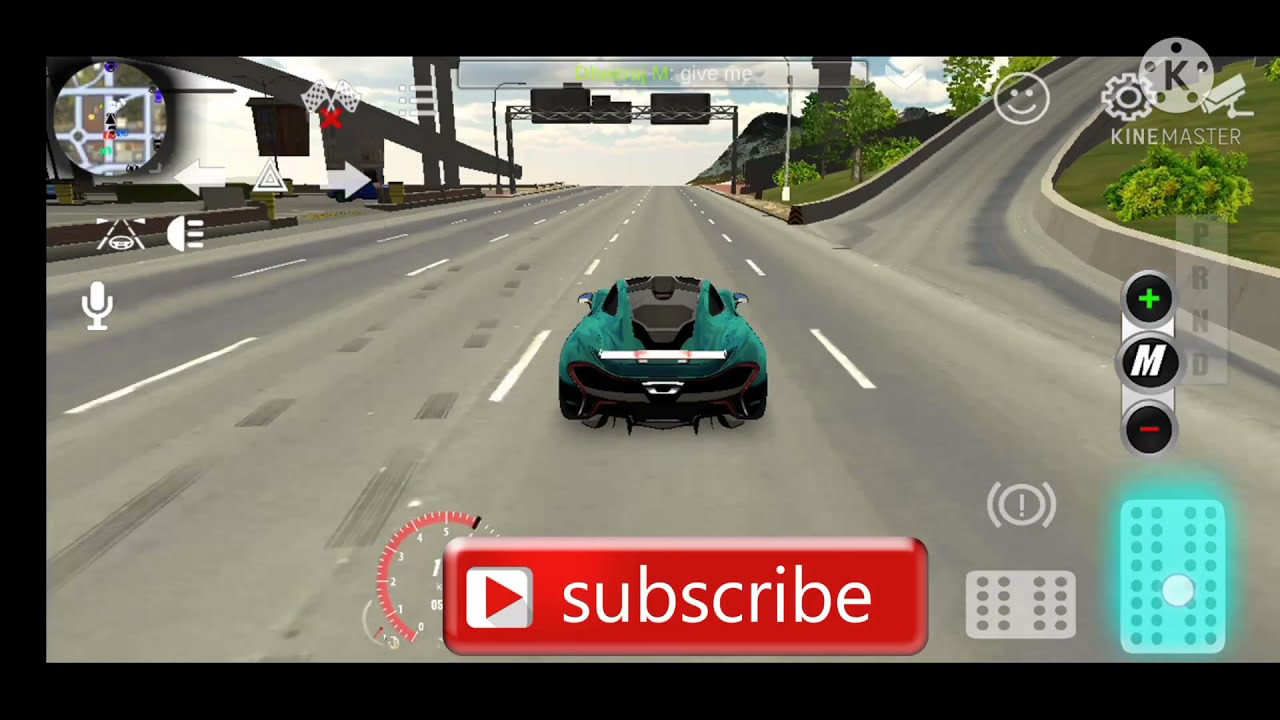This image depicts the splash screen of a computer racing game, presented in a horizontal rectangle with black borders on the top, left, and bottom sides. Dominating the center is a four to five-lane highway receding into the distance. A teal green racing car, parked in the second lane from the right, features distinctive elements such as a black vent or spoiler at the back and some unreadable white lettering across its rear. The car is seen from behind, evoking a sense of depth as it drives away from the viewer.

The upper left corner of the image showcases a navigation circle, while a short wall and several poles parallel the racetrack. In contrast, the upper right corner is crowded with icons: a settings gear, a smiley face, and a light gray circle with a "K" in it, part of the "KineMaster" logo, printed in white text underneath. Vertically aligned below this logo are three black circles marked with a green plus, a white "M", and a red minus, juxtaposed with other white icons of unspecified functions.

The lower middle section hosts a prominent red subscribe button with white lowercase text and a white box with a red triangle to its left. Flanking this button on the left is a partially visible odometer or speedometer. On the right side, a vertical rectangular box encases unfamiliar icons. Further down, a neon blue icon with a glowing outline and additional white game controllers occupy the lower right corner.

In the distance, atop the highway, two overhanging metal trusses support several billboards or signs, hazily leading into the horizon beneath a sky filled with puffy white clouds. To the right of the highway, an off-ramp ascends, bordered by grassy areas and a shrub. This intricate scene combines racing dynamics with an array of game interface elements, drawing players into a vivid, interactive experience.